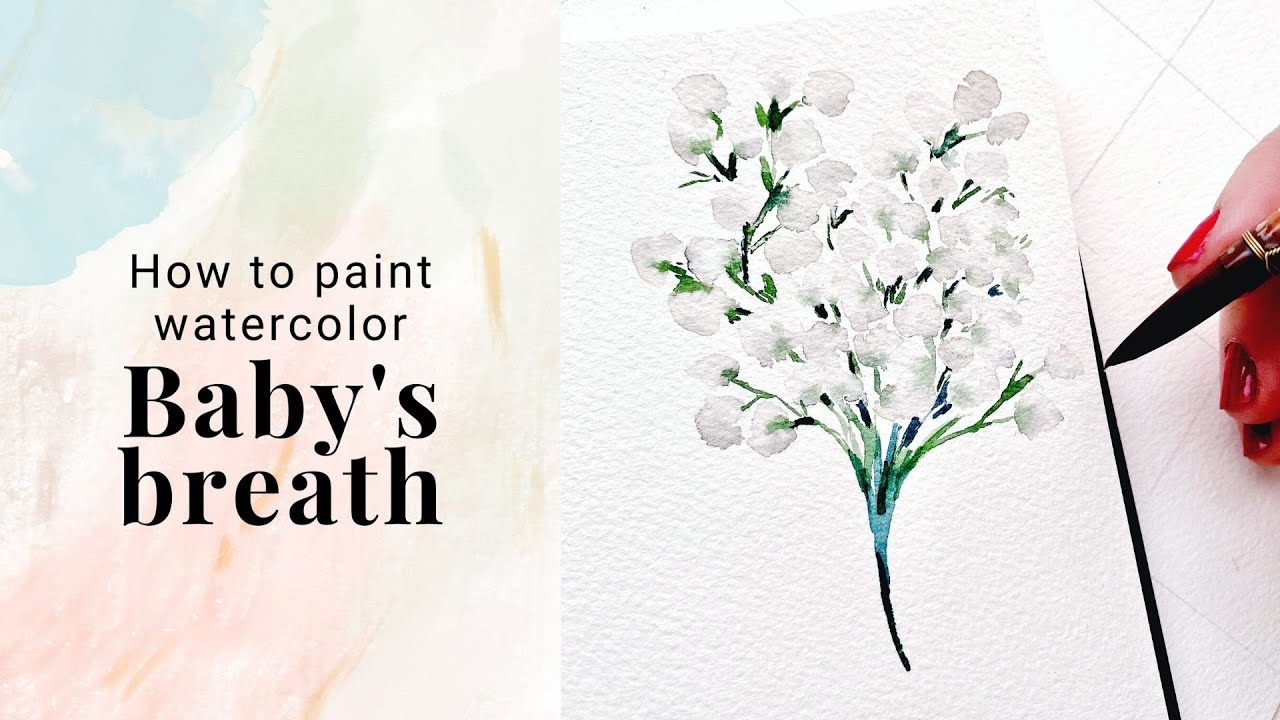The image features an instructional illustration on a white background with the text "How to Paint Watercolor Baby's Breath" in dark lettering. The text is set against a light blue watercolor wash. To the right of the text, there is a detailed watercolor depiction of a baby's breath plant, characterized by clusters of small white flowers connected by dark green stems and highlighted with touches of blue and black. Below the flowers, the stems converge into a pronounced black line. A woman's hand with red nail polish is seen from the left, holding what appears to be a black felt-tip pen, delicately drawing the plant on white paper. The setting is clean and minimalistic, emphasizing the tutorial aspect of painting baby’s breath in watercolor.